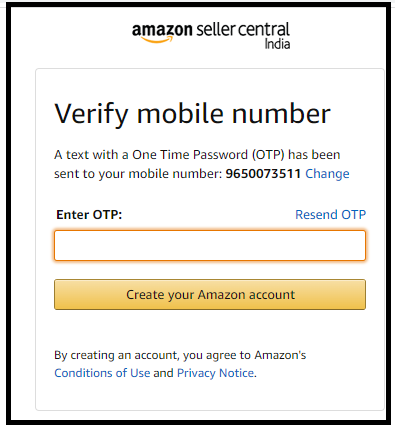The image is a screenshot from the Amazon Seller Central website. In the center of the image is a square box with a black border. At the top center of this box, it says "Amazon Seller Central," and below the word "Central," the word "India" appears in smaller text. 

Beneath this, there is a gray outlined box with bold black letters that say "Verify Mobile Number." Below this header, there is a sentence that reads, "A text with a one-time password (OTP) has been sent to your mobile number: 965-00-73511." The word "change" is displayed in blue next to the mobile number.

Further down, the text "Enter OTP:" is shown in black, followed by a long white rectangular input box with an orange border. On the top right side of this input box, the phrase "Resend OTP" is displayed in blue.

Below the input box, there's a yellow rectangular button with a black border. Inside this button, it says "Create your Amazon account." 

At the bottom of this section, it states, "By creating an account, you agree to Amazon's conditions of use and privacy notice," where "conditions of use" and "privacy notice" are hyperlinked in blue, indicating that they can be clicked for more information. All other words in this sentence are in black.